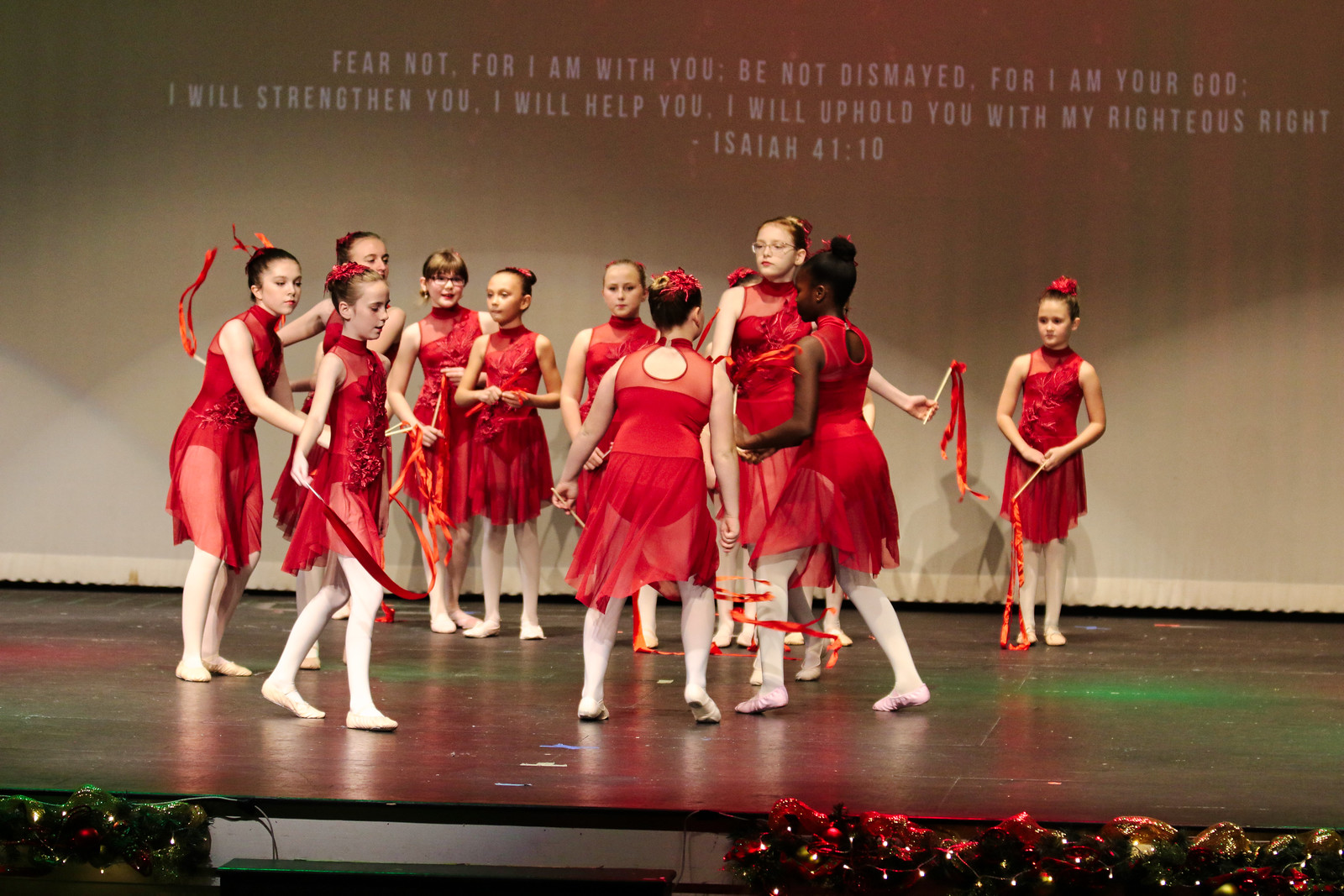The image captures a festive stage set for a Christmas-themed performance. The stage features a wooden floor bordered with garland and Christmas lights, with a step leading up to it. In the background, there is a tan curtain bearing a white projection of a Bible verse, "Fear not, for I am with you, be not dismayed, for I am your God. I will strengthen you, I will help you, I will uphold you, with my righteous right. Isaiah 41:10." 

Front and center on the stage is a group of ten young girls, all dressed in identical long red dresses paired with white stockings and ballet slippers. Their hair is styled in buns, each adorned with red ribbons, and some of them are twirling red ribbons attached to sticks. The girls, who include both white and one black child, with one of them wearing glasses, are positioned in a circle, and appear to be in a moment of pause or preparation during their dance recital. The scene exudes a warm, holiday spirit, accentuated by the red and green lights at the front of the stage.